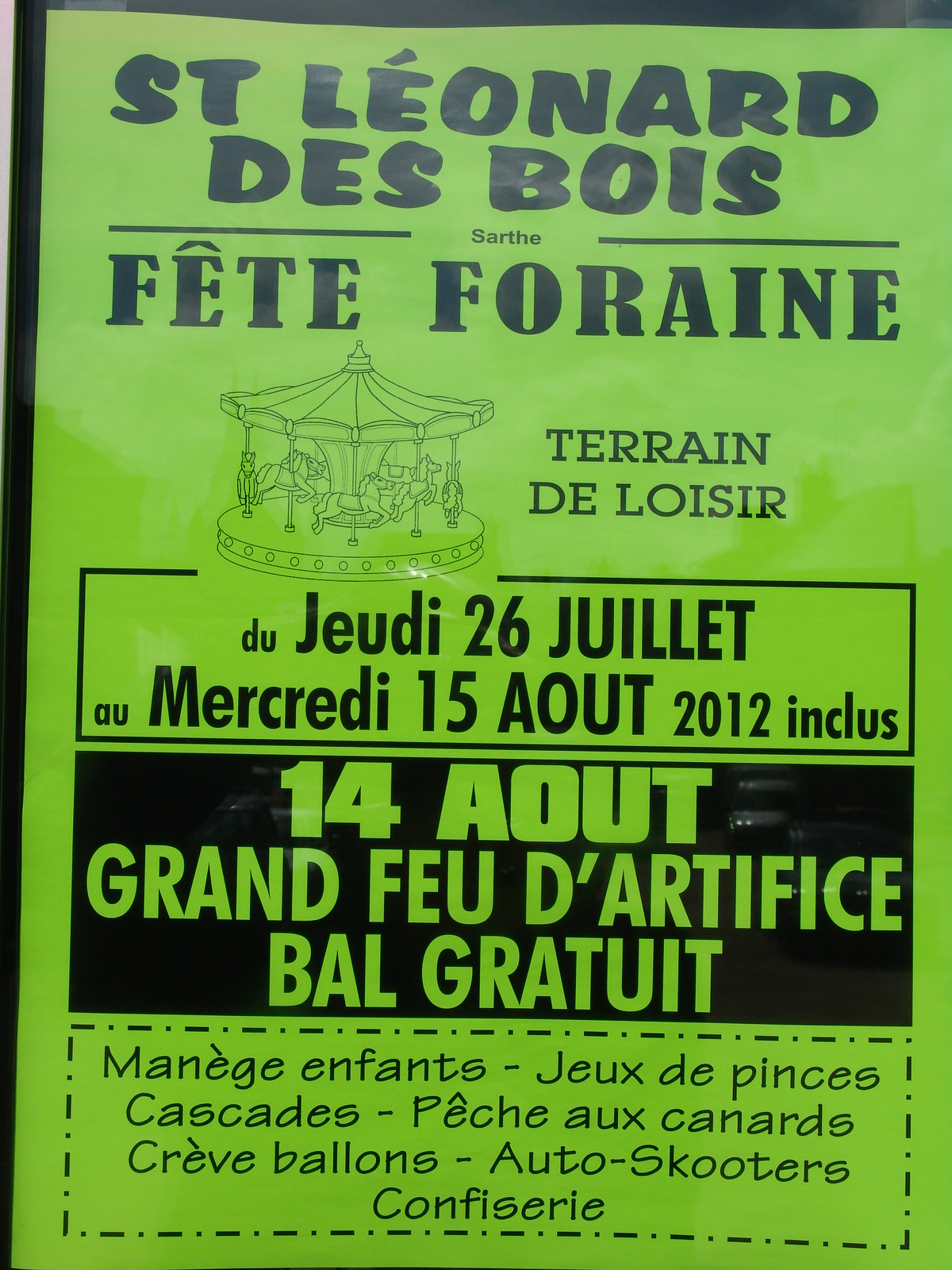Flyer Description: 

The flyer is an eye-catching neon green sheet with bold black text advertising an exciting local event. At the top of the flyer, in large black letters, it reads "ST. LEONARD DES BOIS." Below this is a double black line, and centered between these lines is the word "SARTHE." Further down, in equally bold black text, it announces "FÊTE FORAINE." Accompanying this festive announcement is a stylized drawing of a merry-go-round with horses, positioned on the left side of the flyer.

To the right of the illustration, it reads "TRAIN DES LOISIRS." Additionally, the flyer provides crucial details for the event, stating "du VENDREDI 26 JUILLET au MERCREDI 15 AOÛT 2012 inclus" and announcing a special event on "le 14 AOÛT: Grand Feu d'Artifice."

The bottom section of the flyer features a cutout coupon offering various fun activities and treats, which include "Manège Enfants, Jeux des Pinces, Cascades, Pêche aux Canards, Clé de Ballons, Auto-Scooters," and "Confiserie," ensuring there is something for everyone to enjoy at this vibrant community fair.